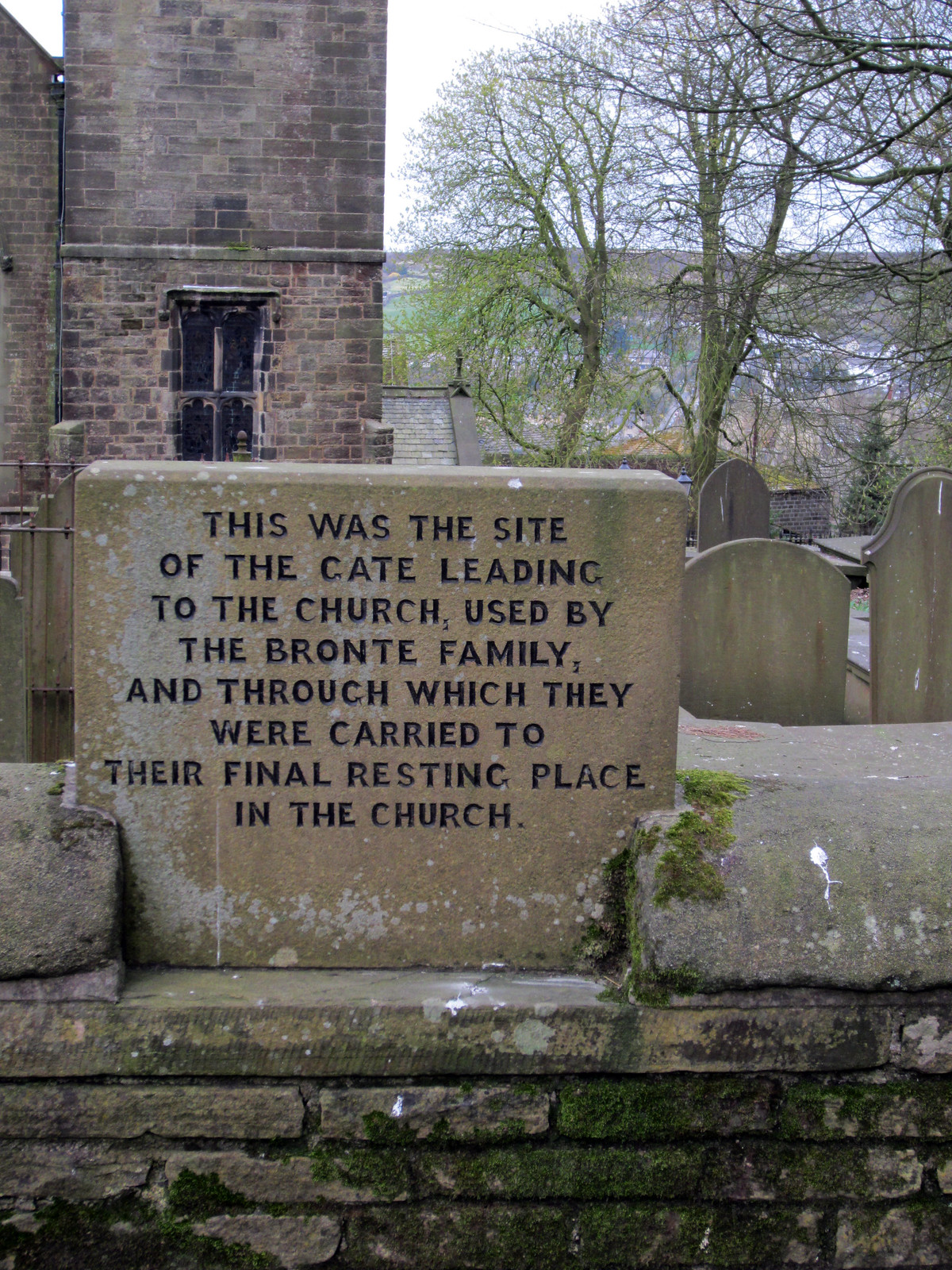This photograph, presented in portrait layout, captures a historical, old piece of architecture with a primary focus on a prominently carved stone sign. The sign, which is roughly two to three inches thick and made of cement, is placed on a small, moss-covered brick wall. Displayed in all capital, serif-style black font, the inscription reads: "This was the site of the gate leading to the church used by the Bronte family and through which they were carried to their final resting place in the church."

The background reveals a scene enriched with history; there's an old, somewhat dilapidated brick building on the left with a window. Further behind the sign on the right, one can glimpse a sky dotted with thin-branched trees, sparse in leaves. Additionally, more gravestones can be observed under these trees, alongside rooftops of further structures and some distant landscape. This comprehensive image offers a detailed snapshot of a site marked by its historical significance to the Bronte family, integrating the solemn gravestones and surrounding foliage.